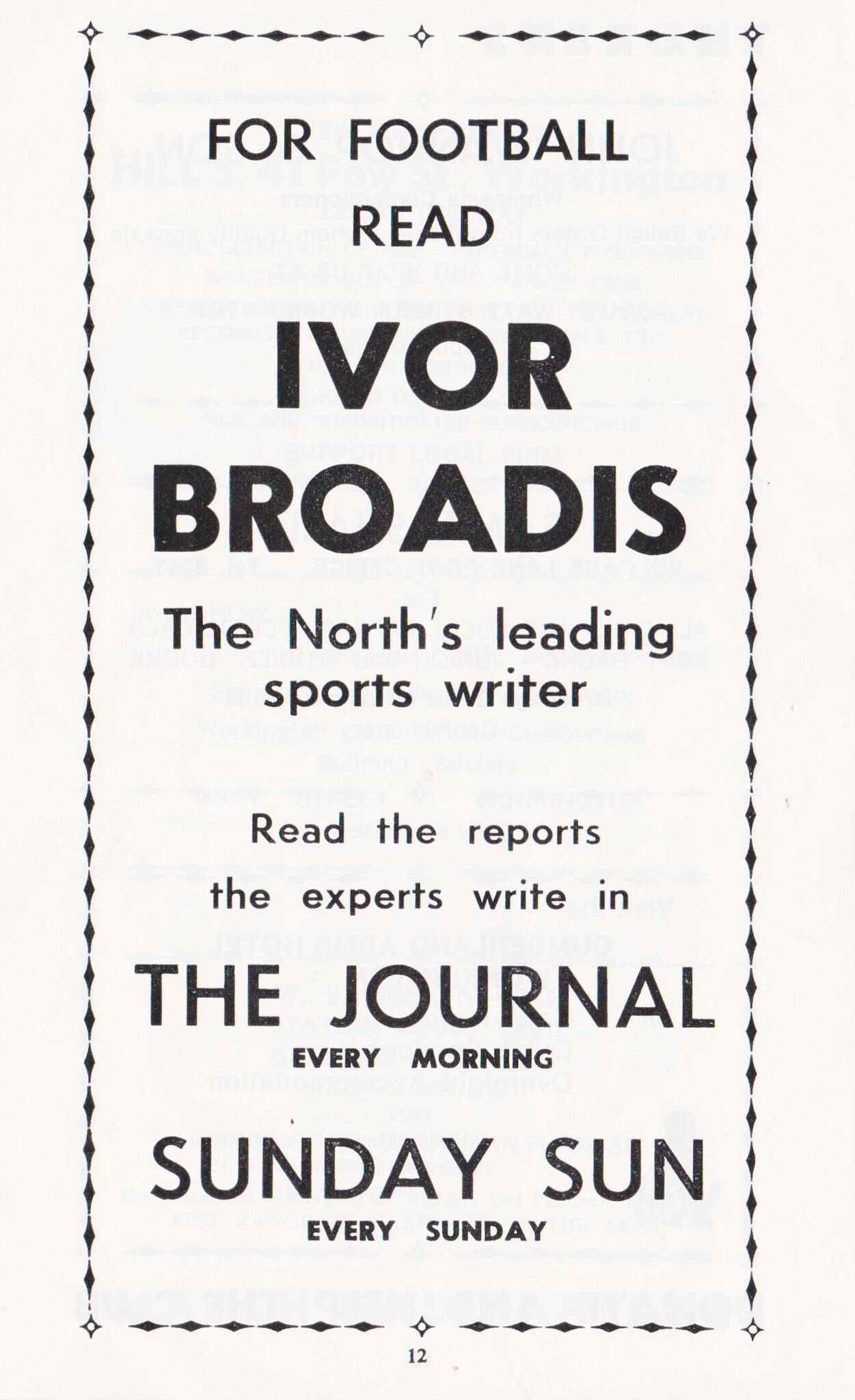The image is a rectangular, portrait-oriented newspaper ad bordered with a diamond-shaped dashed line. In the corners and the middle of the top and bottom borders, larger diamond shapes are present. The centerpiece of the ad proclaims, "For football, read Ivor Broadus, the North's leading sports writer. Read the sports the experts write in The Journal every morning, Sunday Sun every Sunday." The background is white with black text, and a small number "12" is located at the very bottom, suggesting its placement on page 12. The ad promotes Ivor Broadus's football coverage, highlighting his expertise and regular contributions to The Journal and Sunday Sun. The text appears slightly faded, printed on traditional newspaper paper.